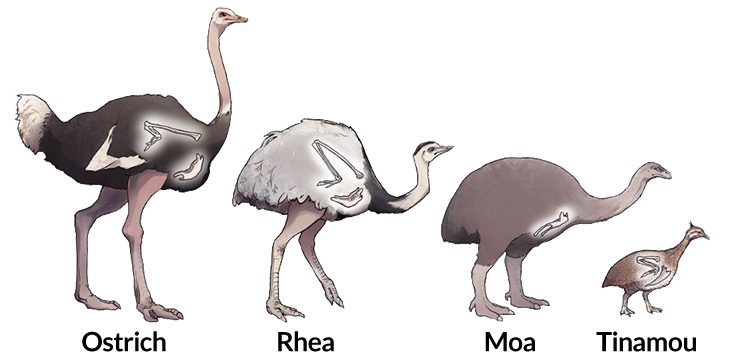The image exhibits four large birds arranged from left to right against a pristine white background, rendering them as if suspended in a void. Each bird is labeled with its name in black text below them, starting with the ostrich on the far left, displaying its notable long pink legs, pink neck, and a rounded bill, alongside a brown body adorned with white feathers on the tail and wings. Next is the rhea, characterized by its long white legs, white feathered body, and a uniquely downward-arching neck topped with a small head and sharp beak. Following the rhea is the moa, distinguished by its stocky legs, entirely brown feathered body, and the absence of wings. Finally, on the far right is the tinamou, illustrated as a small pigeon-like bird with a compact body, short neck, and wings, differentiating itself significantly in shape and size from the others. The organized, linear arrangement of these birds against the monochrome backdrop suggests an educational context, perhaps illustrating evolutionary lineage or diverse avian species profiles.